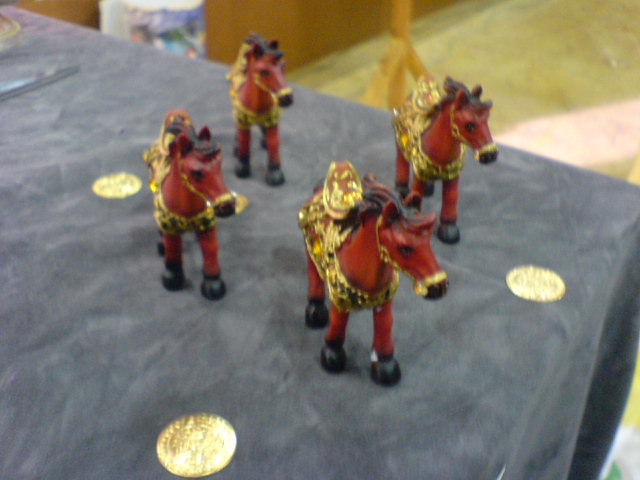This color photograph features four miniature horse figurines, each meticulously aligned and facing the same direction. The horses, colored a rich, brownish-red, boast black hooves, black noses, and black manes. They are adorned with elaborate, shiny gold saddles and bridles, adding a touch of grandeur to their appearance. These figurines rest on a table draped with a light gray tablecloth that appears to be made of a velvet-like material. Scattered around the horses are gold coins that enhance the opulent feel of the scene. In the softly blurred background, a yellowish floor can be seen, providing a subtle contrast to the foreground elements.